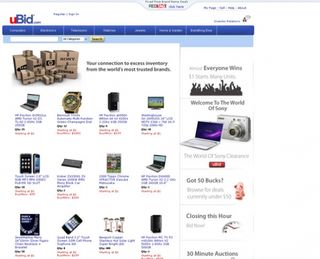This is a detailed screenshot of the website YouBid.com, a platform dedicated to online bidding for various items. Though the screenshot is small and somewhat blurry when zoomed in, key features are discernible. 

At the top of the page, YouBid.com's logo is prominently displayed on the left. The logo consists of a lowercase "u" in red and the word "Bid" in blue, with the first letter "B" capitalized, followed by a smaller ".com" also in blue. Just beneath the logo is a search bar, allowing users to search for items by category.

To the right, near the top of the screen, there's a slogan stating "Everyone Wins," emphasizing the platform's user-friendly experience. Below the search bar, in a blue square, are buttons that categorize the different types of items available, such as laptops, watches, phones, outdoor lighting, video games, and gift cards.

Further down the page, a section hints at an option for users to send their items in, though the details are unclear due to blurriness. Below this section, various item listings are visible, each with its own bidding box. These boxes display items currently available for auction and likely include information on the remaining time for each bid, although the specifics are difficult to read.

Overall, the screenshot captures the essence of YouBid.com as a versatile and user-centric auction site.